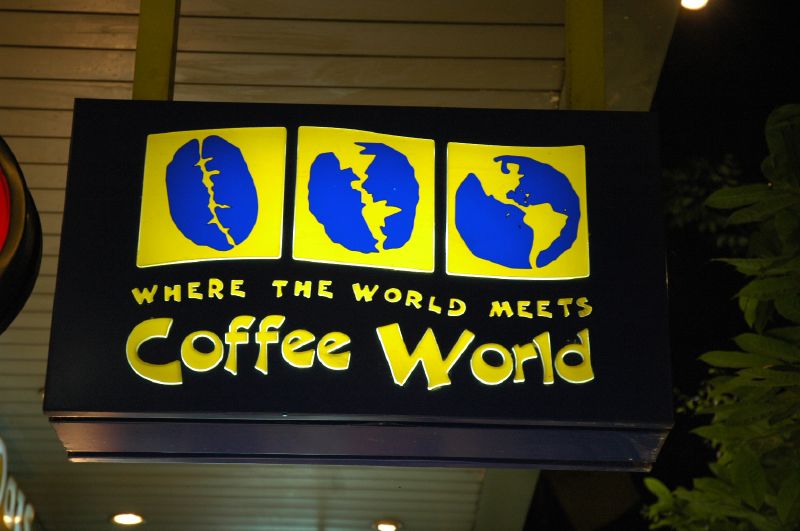This image features an artistic and creative sign for a coffee shop, hanging from the wooden-panel ceiling of an overhang, likely part of a walkway. The scene is dark, suggesting it’s either very early in the morning or at night. The sign, centered in the picture, is a black rectangular prism, crafted from wood or metal. It has three yellow squares with blue drawings: the left one depicts a coffee bean, the right one shows a globe, and the middle square illustrates a transitional phase where the coffee bean morphs into a globe. Below these images, in playful yellow lettering, it reads, "where the world meets," followed by "coffee world" in larger, bold text. Foliage from a tree is visible on the right side of the image, and the bottom of the picture reveals parts of two ceiling lights. Additionally, the left edge of the frame captures a partial view of another sign, which is black with hints of gold and red, but its text is obscured.